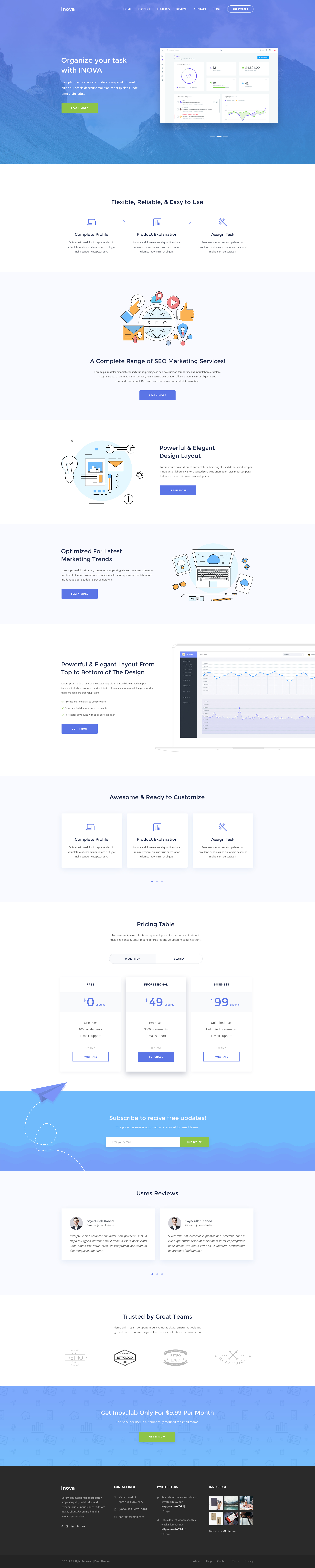The image captures a full-length screenshot of a website, showcasing all its sections in a single view. Due to the scale, the text is largely unreadable, but here is a detailed breakdown of its layout from top to bottom:

1. **Top Section (Header):**
   - A semi-transparent blue rectangular banner occupies the top with what appears to be an overlay of rolling hills.
   - **Left:** A small, difficult-to-read white logo.
   - **Right:** A white navigation menu.
   - **Center-Left:** Text, possibly saying "Organize your tasks with NOVA" (uncertain due to small text size). Below it, there’s a small paragraph in white text and a green button with white text.
   - **Right:** An image resembling an analytics dashboard with various metrics.

2. **First White Section:**
   - **Heading:** Appears to read "Flexible, Something Remarkable, Easy to Use."
   - Below are three points, each featuring icons, titles, and brief paragraphs, which are too small to read.

3. **Light Gray Section:**
   - **Graphic:** A central circle surrounded by app icons (thumbs-up, play button, location service, mail, and a finger-pointing app).
   - **Text:** "Complete something of marketing services" followed by a short paragraph and a blue button with white text.

4. **Second White Section:**
   - **Illustration:** Possibly a computer monitor displaying a bar chart.
   - Icons to the left: light bulb, envelope, pencil, and wrench.
   - **Right:** Black heading, a paragraph, and a blue button with white text.

5. **Gray Section:**
   - **Right:** An image of a laptop accompanied by sunglasses and a desk photo.
   - **Left:** Black heading, a small paragraph, and a blue button with white text.

6. **Third White Section:**
   - **Left:** Heading, a paragraph with bullet points, and a blue button with white text.
   - **Right:** Graphic of a line chart remaining level.
   
7. **Third Gray Section:**
   - **Heading:** Black text.
   - Below: Three information boxes, each with an icon, bold heading, and a paragraph.

8. **Fourth White Section:**
   - **Heading:** Black text.
   - Details on pricing tiers:
     - **Left:** $0 plan with a list of features.
     - **Middle:** $49 plan highlighted, with a blue button.
     - **Right:** $99 plan with features listed.
   
9. **Blue Section (Email Subscription):**
   - **Heading:** White text.
   - Paragraph and an email input box with a green button.

10. **Light Gray Section (User Reviews):**
    - **Heading:** "User Reviews."
    - Two blocks with avatar images, names, job titles, and reviews.

11. **Final White Section:**
    - **Heading:** "Trusted by something teams."
    - A few sentences followed by various business icons.

12. **Final Blue Section:**
    - **Heading:** White text and a green button with white text.

13. **Footer (Black Section):**
    - **Columns:**
      - **Left:** Company information with white headings and details.
      - **Right:** A collage of very small product images.

This comprehensive layout reveals a professional, multi-faceted website that focuses on task organization and marketing services, featuring modern design elements, diverse sections for various types of content, and clear call-to-action buttons throughout.